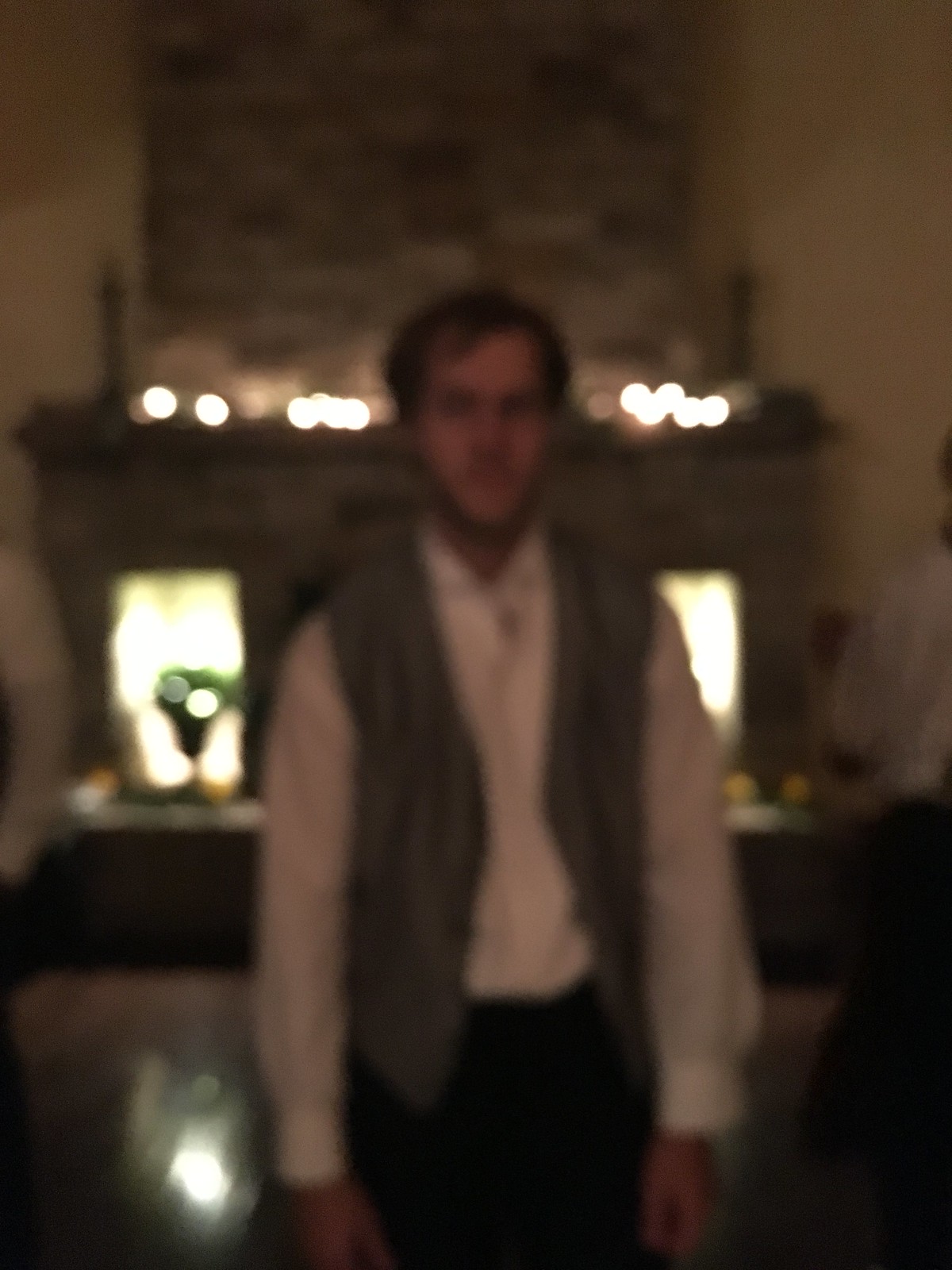In this sepia-toned, out-of-focus photograph, a man with short dark hair and a serious expression stands on a hardwood floor in front of a stone brick fireplace adorned with string lights. He is dressed in a white long-sleeve, unbuttoned collared shirt with lengthy cuffs, and a gray vest that V's in and out, complemented by dark pants. His arms hang at his sides, and behind him, the fireplace mantel is decorated with candles and candlesticks. To the left of the image, there appears to be a piece of furniture, possibly with a sewing machine on top, set in front of a window letting in light. The scene is blurred and pixelated, yet it evokes an old western aura, highlighted by the man's attire and the vintage ambiance of the surroundings.